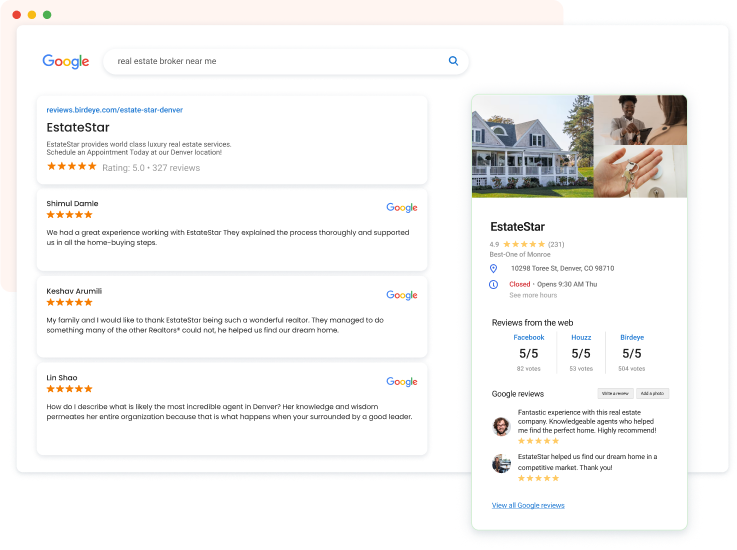This is a detailed screenshot from a Google search results page for "real estate broker near me." The layout shows a light pink border on the left side covering about two-thirds of the height and a matching border across the top covering about three-quarters of the width. The bottom and right sections are white. 

In the top-left corner within the pink border, there are three colored circles: red, yellow, and green, typical of a browser's window controls. Below that, the background is white.

The search interface features the iconic multicolored "Google" logo in the upper-left corner, with a search bar extending halfway across the page displaying the search phrase "real estate broker near me" in black text. To the right of this search bar is a blue search icon. Below this bar, there appear to be several review entries formatted in a stacked layout:

1. **First Review Entry**:
   - **URL**: "birdies.com/estate-star-denver" in blue text.
   - **Title**: "Estate Star" in bold lettering.
   - **Details**: Two lines of informational text.
   - **Rating**: Five stars, with a text notation "5.0" and "327 reviews" next to the stars.

2. **Second Review Entry**:
   - **Title**: Name of the establishment, followed by five stars.
   - **Details**: Two lines of informational text with "Google" in the top-right corner.

3. **Third Review Entry**:
   - Similar format to the second entry with the name, five stars, and Google's logo in the corner, along with two lines of informational text.

4. **Fourth Review Entry**:
   - Same structure as previous entries but with a slight variation in the positioning of Google's logo.

On the right side of the page, there's a pop-up tab featuring real estate information:
   - **Top Third**: Contains two images. On the left, there's a photo of a gray house with a blue roof, a tree on the right, and a grassy lawn. On the right, there's an image of an African American woman handing keys to another woman whose back is to the camera.
   - A smaller image below shows a hand holding keys.
   - **Title**: "Estate Star" in bold black letters.
   - **Rating**: Displayed prominently with star icons.
   - **Address** and operational hours.
   - **Reviews from the Web**: Includes sources like Facebook, Hours, and BirdEye.
   - **Google Reviews**: Two individual reviews listed.
   - At the bottom, a blue, underlined link reads "View all Google reviews," indicating a clickable option to see more reviews.